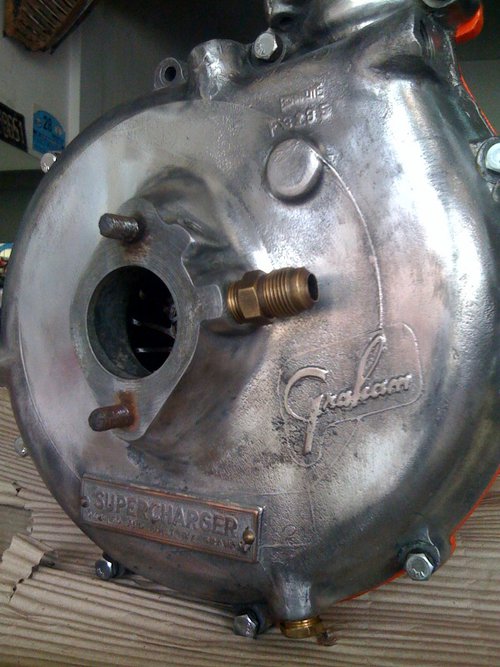The image captures the front view of a large, heavy metal object, specifically a supercharger, prominently positioned in the center against a backdrop of a garage or workshop. The supercharger, composed mainly of silver metal with various bolts protruding, features a notable gold attachment at its center for hose connections, and a central cutout flanked by two bolts. At the bottom of the device, within a rectangular outline, the word "SUPERCHARGER" is embossed in all caps, accompanied by other unreadable text below. The background shows white walls, a metal sign, and possibly a license plate. The supercharger rests on light brown, slightly torn and rippled cardboard. Colors in the photograph include silver, gold, light blue, yellow, red, and shades of brown and tan, with a hint of red wear at the top right of the machine.